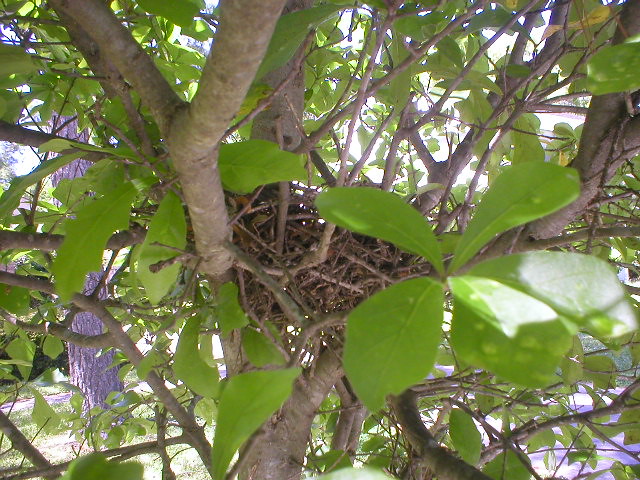In this vibrant photograph, a bird's nest, crafted from an intricate network of twigs and nestled perfectly amidst the branches of a mature tree, takes center stage. The tree's branches exhibit a variety of thicknesses and hues of brown, creating a complex and textured foreground. Surrounding the nest, numerous teardrop-shaped leaves in shades of green, some speckled with lighter green or yellowish spots, sprout generously from the branches. The sunlight filtering through the foliage creates a mesmerizing pattern of light and shadow. The bright summer sky peeks through the gaps between the leaves and branches, contributing to the overall warm and serene atmosphere. Despite the nest’s empty state, the scene exudes life and tranquility, amplified by the occasional yellowing leaf, indicating the subtle transitions of nature. In the top corners of the image, parts of the sturdy tree trunk and additional branches can be seen, grounding the scene in its natural, lush setting.